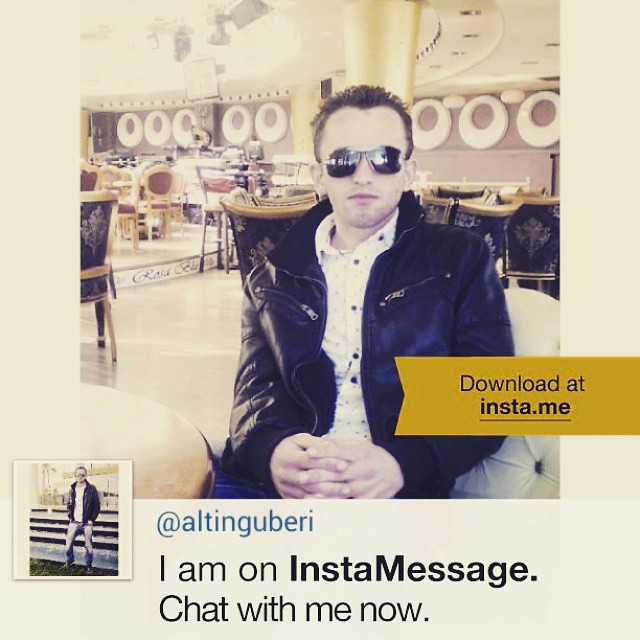The image features a man of Caucasian descent sitting in an ornate dining area, possibly a restaurant or an event center. He is wearing a black leather bomber jacket, unzipped to reveal a white button-down shirt, and has short spiky brown hair with a receding hairline. His dark sunglasses obscure his eyes as he looks directly at the camera with a serious expression, his hands clasped in front of him. The setting is elaborate, with elegant chairs that have black and gold trim and some with burgundy and gold upholstery. The background includes large golden poles and circular white decorations on the walls, contributing to the sophisticated ambiance.

On the right-hand side of the image is a gold banner with the text "download at insta.me" in black print, underlined. Below it, in blue font, is "@AltonGuberi." Additionally, there's a message inviting viewers to chat, stating, "I am on insta message. Chat with me now."

Inset in the lower left corner of the image is a smaller photo of the same man. In this snapshot, he is standing, dressed in the same black jacket and white shirt, paired with blue jeans. The background of this smaller photo is somewhat ambiguous, possibly an outdoor setting with a structure resembling an animal pen or a fountain.

The main photograph is bordered in a light tan, almost yellowish shade on the left, right, and bottom, accentuating the image's overall composition.